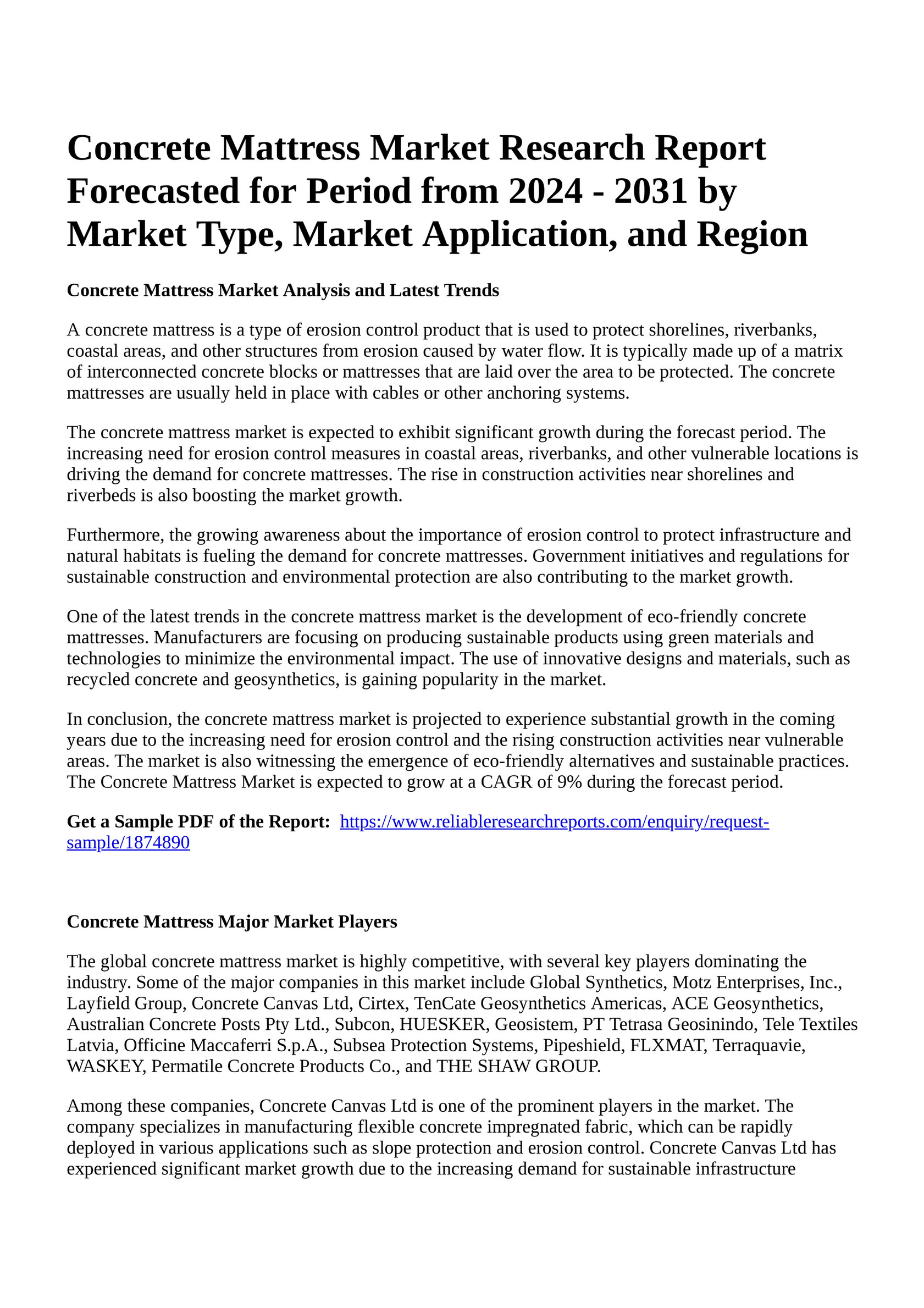The image depicts an online article titled "Concrete Mattress Market Research Report, Forecasted for the Period from 2024 through 2031 by Market Type, Market Application, and Region", written in bold black text at the top. Beneath this title, also in bold, are the words "Concrete Mattress Market Analysis and Latest Trends". The article explains that a concrete mattress is an erosion control product designed to protect shorelines, riverbanks, coastal areas, and other structures from water-induced erosion. The body of the text is unindented and separated by spaces between paragraphs. Midway through the article, there's a bold black line of text reading "Get a Sample PDF of the Report" followed by an underlined blue link. Further down, another bold heading announces "Concrete Mattress Major Market Players," followed by additional paragraphs listing key companies. The entire article is set against a plain white background and features three main colors: black, blue, and white.